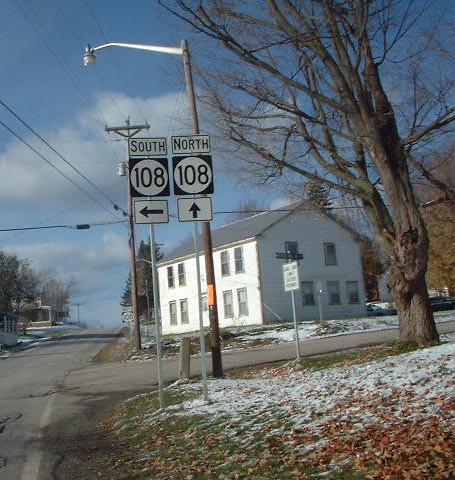This square color photograph captures a small, cracked, one-lane street in a quaint American town, as indicated by the street signs. It's wintertime, with a light dusting of snow on the grassy ground, interspersed with red and brown dried leaves. Dominating the middle of the frame is a large, white clapboard, two-story house with a gray roof. The house has four windows on the upper level and two on each side of a central door on the lower level. A tall, barren deciduous tree stands prominently on the right, its leafless branches contrasting with the overcast blue sky and white clouds.

In the foreground, two vertical street signs on silver poles stand embedded in the grass. The left sign, with "South 108" in black letters on a white circle against a black background, has an arrow pointing left. The right sign similarly reads "North 108," with an arrow pointing straight ahead. In front of these signs is a streetlight, and overhead, telephone wires stretch across the sky. The scene is further enlivened by a large tree to the right and a big pine tree visible behind the house.